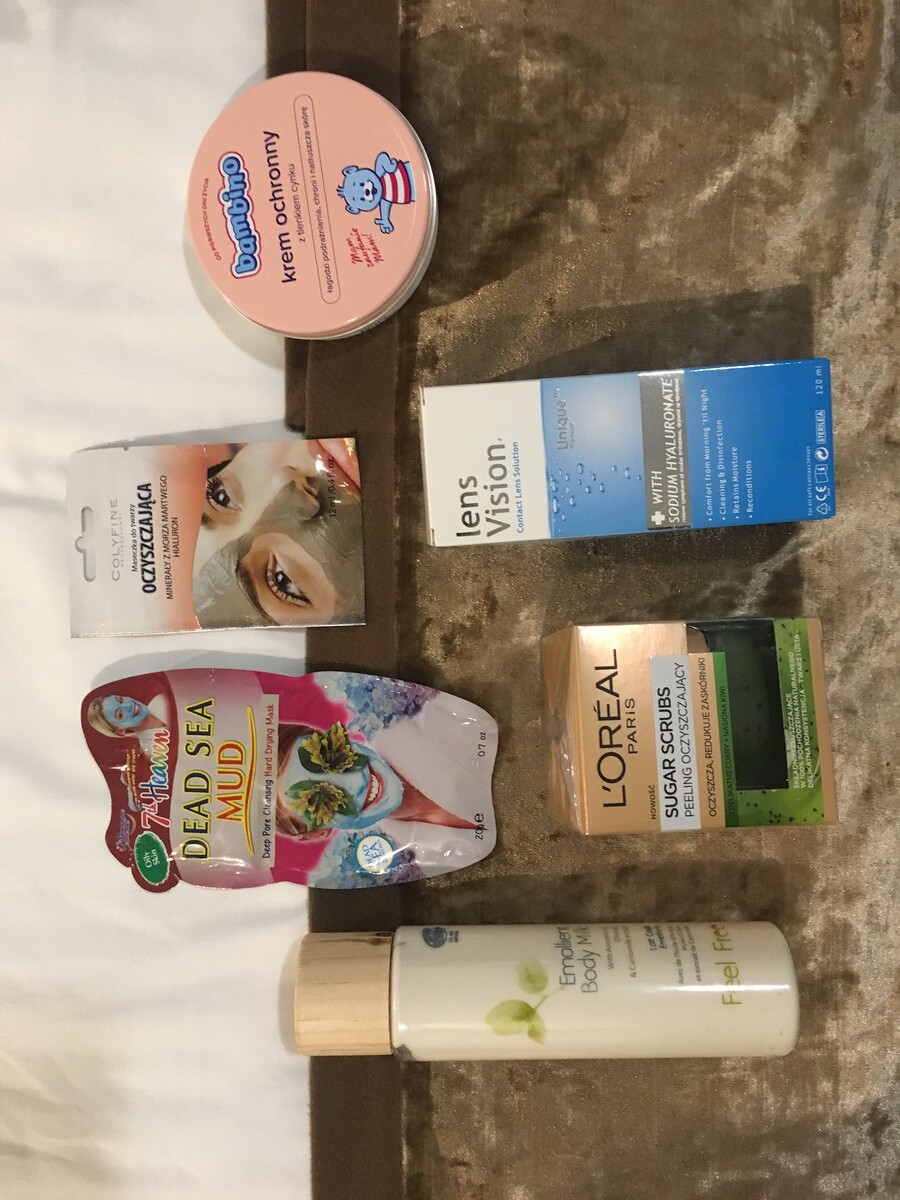The image showcases a countertop in hues of gray and brown, captured from a sideways perspective. On the countertop, several beauty products are arranged. To the far left, there is a long, cylindrical plastic bottle with a bright light brown cap labeled "Emollient Body Mist," adorned with green leaf designs. Adjacent to it is a product labeled "Dead Sea Mud Mask," featuring an image of a woman with a blue mask on her face. Next in line is a jar of "L'Oreal Paris Sugar Scrubs." Additionally, there is another mud mask product displaying an image of a face with mud covering half of it. Near these items, a package labeled "Lens Vision" and a round, flat container marked "Crème Chandrony" are also visible on the countertop.